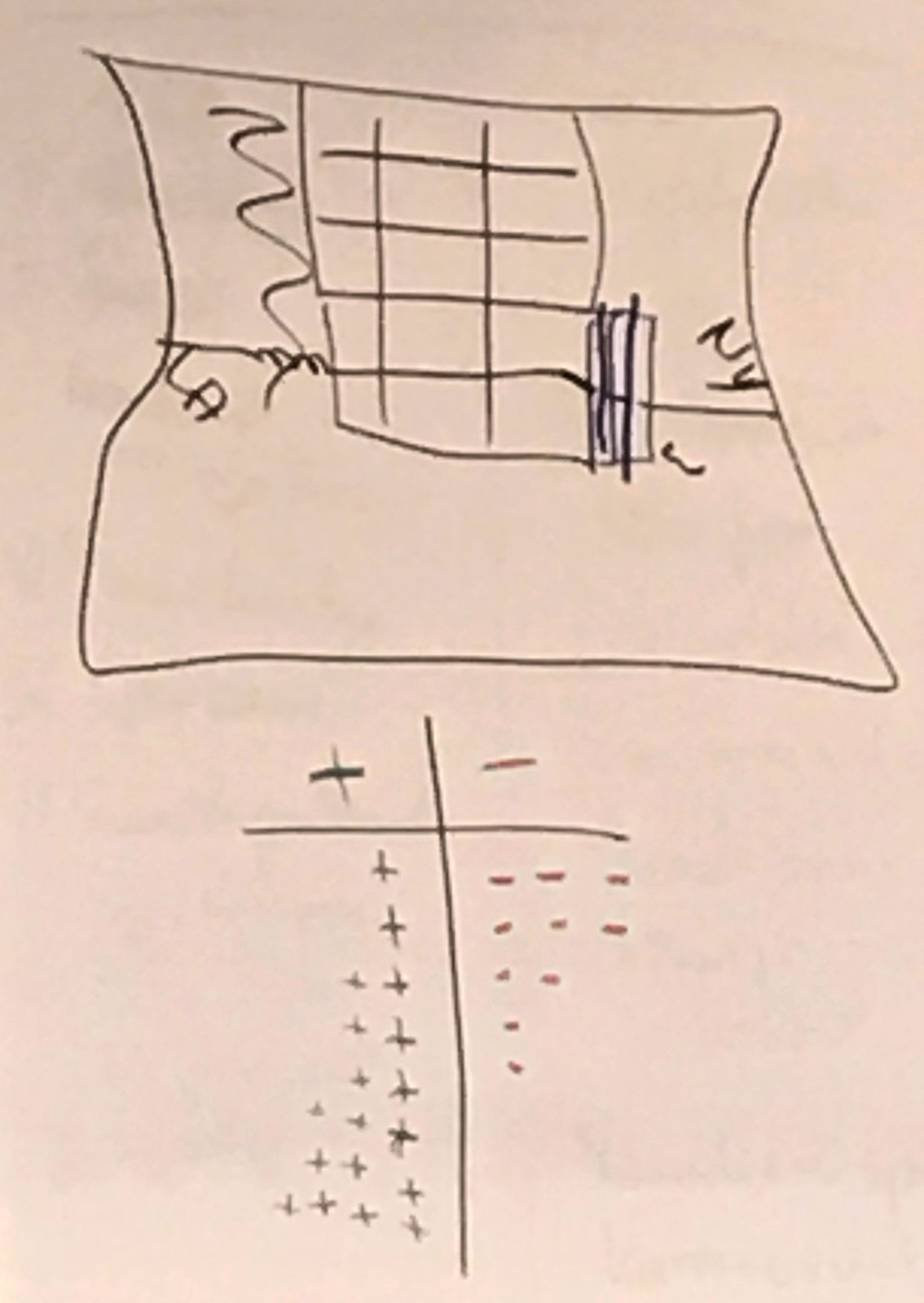The image features a buff-colored piece of paper adorned with a unique, hand-drawn illustration in a broad black pen. Dominating the upper half of the paper is a roughly sketched square bisected horizontally by a somewhat jagged line, reminiscent of a resistor in an electrical circuit. On the right side of this line, within the square, is the label "NY," and on the left is "LA." Nested within the upper part of the square, intersecting the central line, is a smaller rectangle divided into a grid by two vertical and four horizontal lines, resembling an extended tic-tac-toe board.

Below this intricate grid lies a rudimentary score tracking system. At its top is a large cross formed by a vertical and a horizontal stroke, accompanied by a header marked with a plus and a minus sign. Underneath, several rows tally scores using pluses and minuses. The plus column records sequences as follows: one plus, one plus, two pluses, two pluses, two pluses, three pluses, three pluses, and four pluses. The minus column tracks: three minuses, three minuses, two minuses, one minus, and one minus. This setup suggests an ongoing scorekeeping effort for a game or activity, meticulously noting the results in sequential rows.